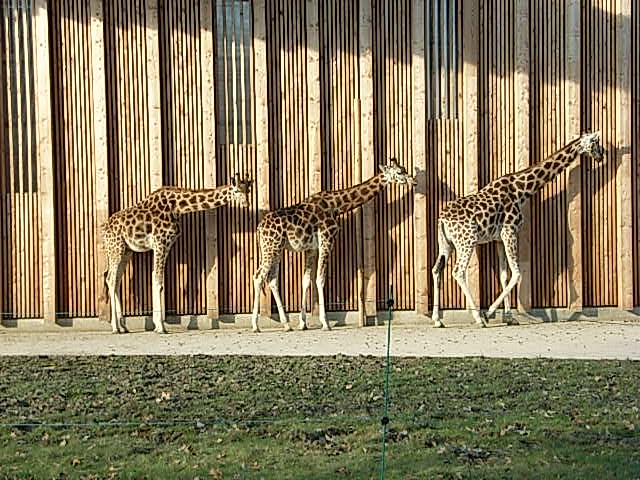This image captures a row of three giraffes walking to the right in what appears to be a zoo enclosure. The giraffes are of varying sizes, with the tallest one leading the group, suggesting it could be a mother with two adolescent or young adult giraffes. The giraffes are situated on a light gray paved pathway and adjacent to an elaborate wall structure. The wall features vertical wooden timbers or slatted bamboo elements and several vertical concrete supports, contributing to a complex pattern of textures. Directly in front of this walkway is a grassy area, dotted with some dry leaves, emphasizing a natural setting, possibly during summertime, given the deep green hue of the grass. The giraffes carry a distinctive yellowish coat with brown spots, along with lighter white legs and feet with black soles. Their shadows cast prominently on the wall behind them suggest a low sun position, either at dawn or dusk. The background also includes a green fence or some kind of wire enclosure, adding to the zoo-like ambiance of the scene.